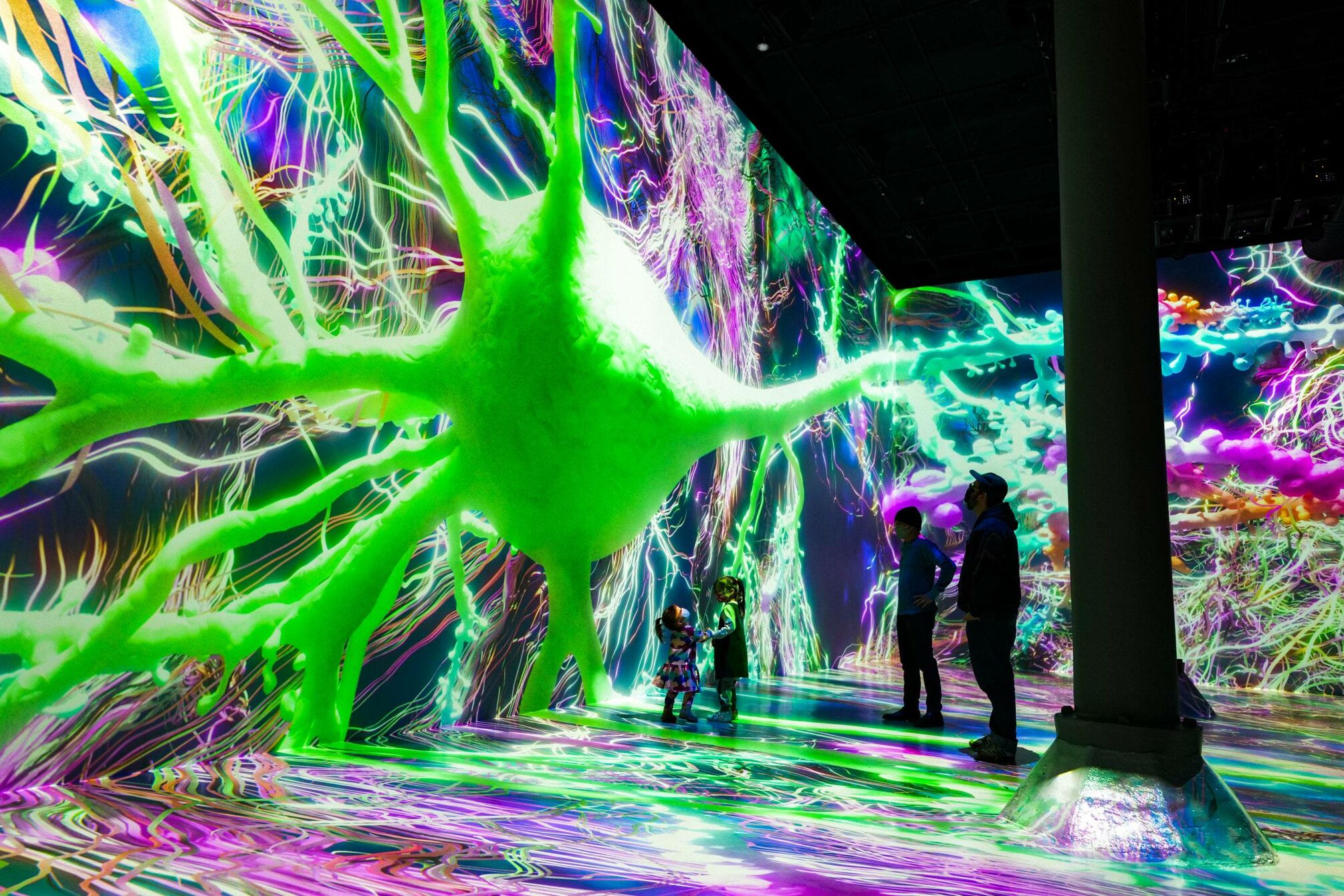The image captures a vibrant art installation, likely taken at an art gallery or interactive exhibition space. Dominating the scene are two vividly decorated walls and a floor splashed with a rainbow of neon lights that resemble scattered paint. A large, green neuron-like structure with dendrites and axons extends across the left wall and even into the right wall, creating a central focus amidst the colorful chaos. The ceiling starkly contrasts with its deep black color, matching the similarly black column on the right side that seamlessly integrates into the floor. Viewing this immersive display are four figures – two adults and two children – who stand awed by the sensory overload of hues including green, purple, blue, and more glow-in-the-dark tones. A tall black pole, which appears to support a light, further illuminates the scene, enhancing the intricate and dynamic light effects.